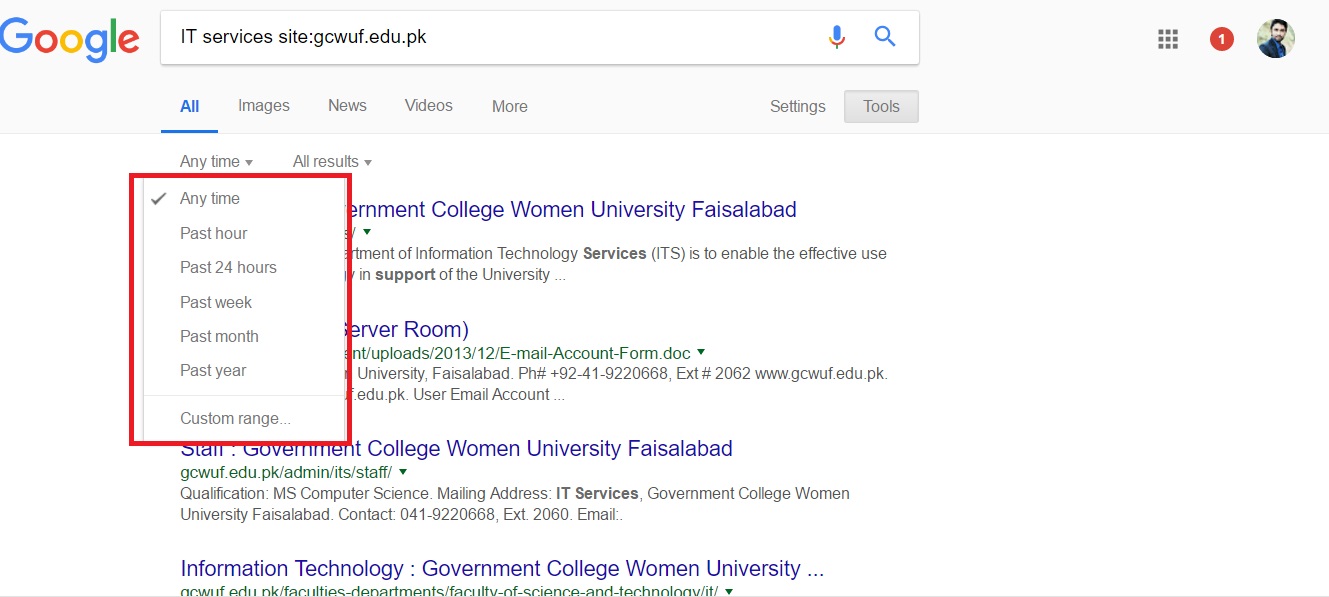This image is a screenshot of a Google search results page. At the top, there is a light gray banner featuring the Google logo on the left side. The logo consists of a capital "G" in blue, followed by a lower-case "o" in red, another "o" in yellow, a "g" in blue, an "l" in green, and an "e" in red.

Below the banner, there is a search bar with the text "IT services site: GCWUF.edu.pk" in black lettering. To the right of the text within the search bar, there is a microphone icon and a magnifying glass icon.

To the right of the search bar within the gray banner, there is a grid of nine small squares arranged in a 3x3 pattern, representing Google's app launcher. To the immediate right of this grid is a red circle containing a white number one, indicating a notification. Further to the right, there is a circular icon displaying a man's picture.

Below the gray banner, there is a navigation bar that includes the categories: "All", "Images", "News", "Videos", and "More". The "All" category is in blue and underlined, indicating it is the currently selected category. To the right of these options, there are links for "Settings" and "Tools", with a rectangular border around "Tools".

The main content area has a white background. Directly under the navigation bar, there is a dropdown menu next to the text "Any type," which lists options such as "Any type," "Any time," "Past hour," "Past 24 hours," "Past week," "Past month," "Past year," and "Custom range." These options are outlined by a red border.

Further down, another dropdown menu labeled "All results" is present, though it partially obscures some underlying text. This dropdown likely provides options for filtering search results based on various criteria.